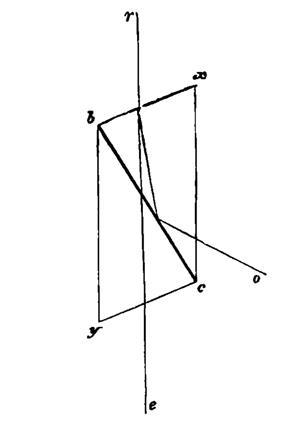The image is a technical-looking line drawing on a white background, showing a rhombus that appears tilted and, thereby, resembles a diamond. Each corner of the rhombus is labeled with various Greek and Latin letters or symbols—one corner is marked as B, another as J, one looks like a lowercase y, and the last one as C. This rhombus is divided diagonally into two isosceles triangles by a gray line stretching from one corner to the opposite corner.

In front of this rhombus, a straight vertical line intersects it from the top, labeled R at the top and lowercase e at the bottom. There is another line forming an obtuse angle that starts from the top middle of the rhombus, intersects the diagonal line, and then extends beyond the bottom edge, creating another endpoint labeled O. Despite the complexity and variety of lines and angles, the figure doesn't explain its purpose or meaning, lending it an air of technicality without clear functional significance. All elements of this diagram, including the black and gray lines and letter labels, contribute to an overall sense of geometric abstraction.